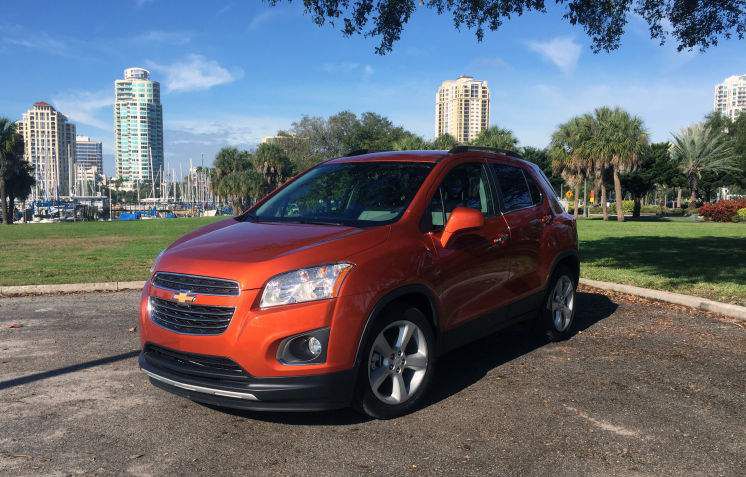The image captures an outdoor setting featuring a small, rust-orange Chevrolet two-door car parked in a neatly paved black parking lot. The car, likely an economy model, is positioned near a white concrete curb that borders a grassy park area. In the background, a scenic view unfolds with a harbor showcasing the masts of sailboats. Further back, a cityscape of tall high-rise buildings in various shades of white, green, and gray contrasts against the vibrant blue sky adorned with only a few wispy clouds. The image conveys a sense of pride in the vehicle while situating it in a picturesque, urban-meets-nature environment.